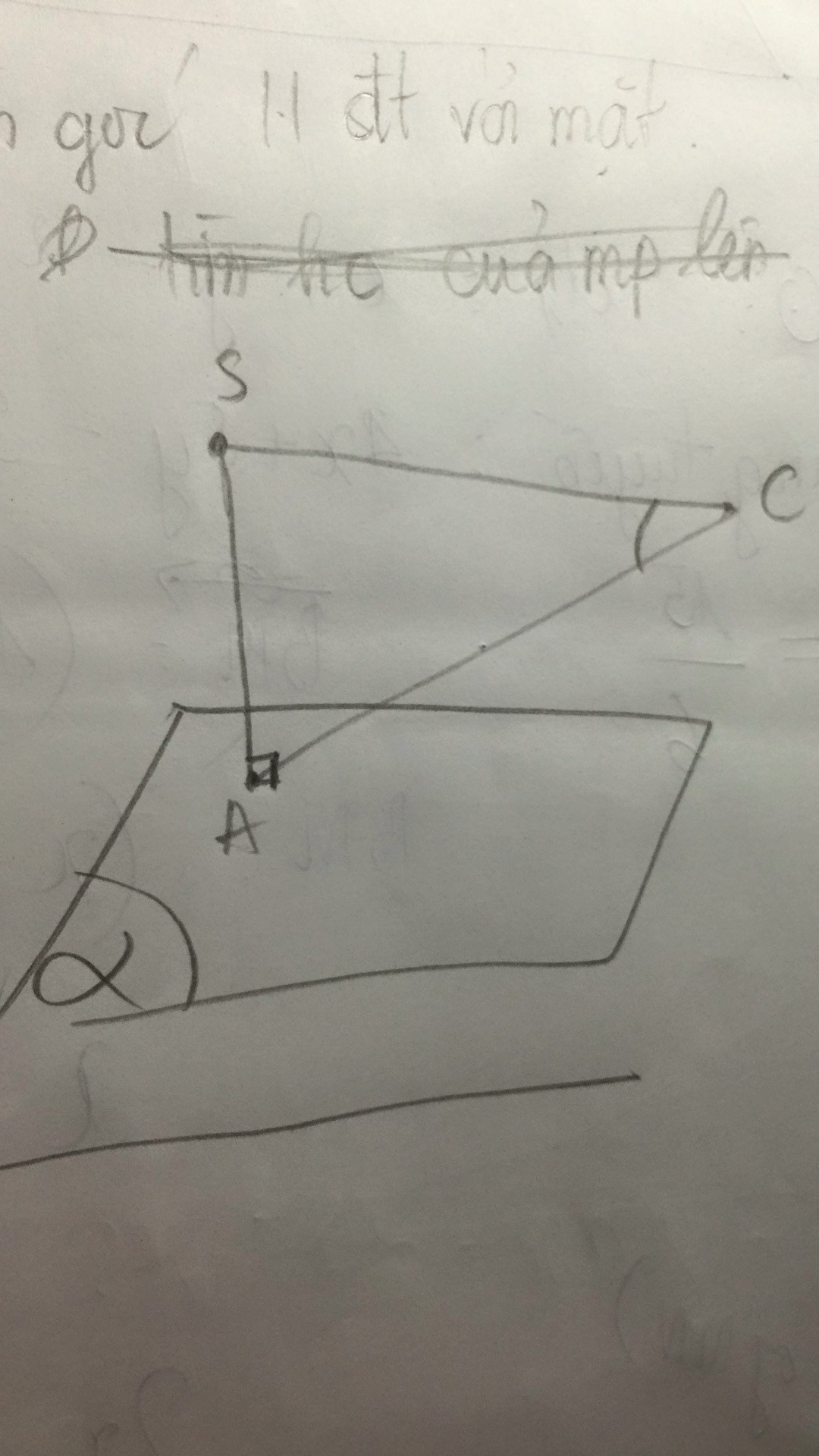This image features a piece of white paper adorned with pencil sketches and notes that appear to be part of a homework assignment. At the top of the page, partially scratched-out writing can be seen, possibly in Spanish, with the words "him, he, qua, m-p-l-e-n" faintly discernible. Below the scratched-out text, there is an irregularly drawn box, tilted slightly to the right. In the lower left-hand corner of this box, a small fish is sketched. 

Overlapping the box is a triangle labeled at its vertices: 'A' at the bottom, 'S' at the top, and 'C' at the right-hand corner. Extending from the bottom left-hand side of the paper and traversing about 80% of the width is a single, straight horizontal line. The bottom 10-15% of the page remains blank, free from any drawings or notes.